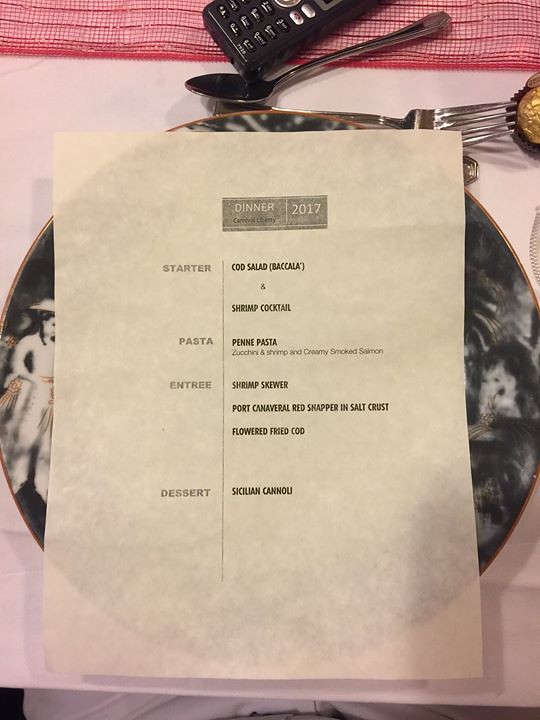A meticulously set dining table is captured in the image. At the upper center of the image lies a portion of a remote control. Below the remote, a spoon is angled to the left, while a fork points to the right. A plate with an intricate, though indistinguishable, design decorates the center of the frame, featuring a subtle white figure on the left side. The plate is partially obscured by a menu detailing a dinner from the year 2017. The menu begins with a choice of a Cobb salad or shrimp cocktail as a starter, followed by a penne pasta course. For the entree, options include a shrimp skewer, red snapper, or cod. Concluding the dinner, Sicilian cannoli is offered for dessert. This scene, seemingly set in a winery or upscale restaurant, exudes an atmosphere of anticipation for a memorable meal.